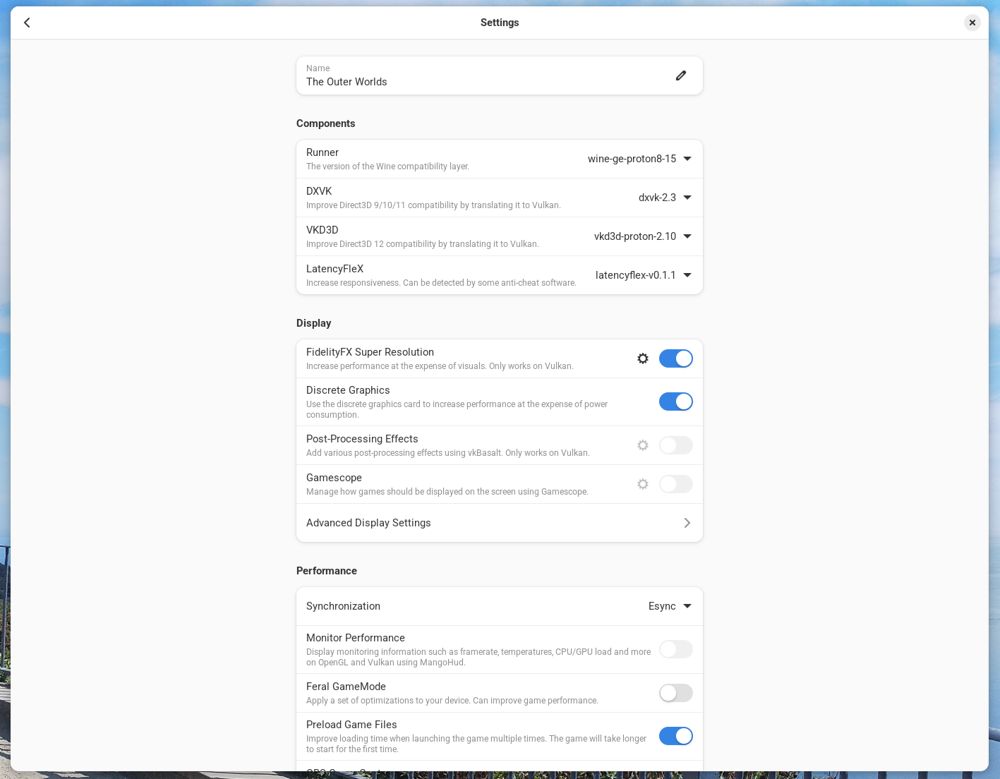This image showcases a detailed settings section of a software application. At the top, a white slider prominently displays the title "Settings". Below this header, the first section labeled "Name the Older Worlds" is followed by a “Components” section. This section lists several components with corresponding drop-down menus: "Runner DXVK," "VKD3D," and "Latency FLEX."

Underneath the components, the "Display" section features various options. Here, "Fidelity FX Super Resolution" is enabled, indicated by a blue slider. Similarly, "Discrete Graphics" is also turned on, shown by another blue slider. However, "Post Processing FX" and "Game Scope" are turned off. An expandable menu titled "Advanced Display Settings" is available, marked with an arrow suggesting additional options can be accessed.

The "Preference" section starts with "Synchronization" which includes an option for "E-Sync" that comes with a drop-down menu. This is followed by a "Monitor Preference" setting, which is currently turned off. Also turned off is the "Farewell Game Mode." Lastly, the "Preload Game Files" option is enabled, as indicated by its blue slider.

Overall, the image illustrates a comprehensive and customizable settings interface with various toggles, drop-down menus, and expandable sections for fine-tuning the application’s performance and visuals.